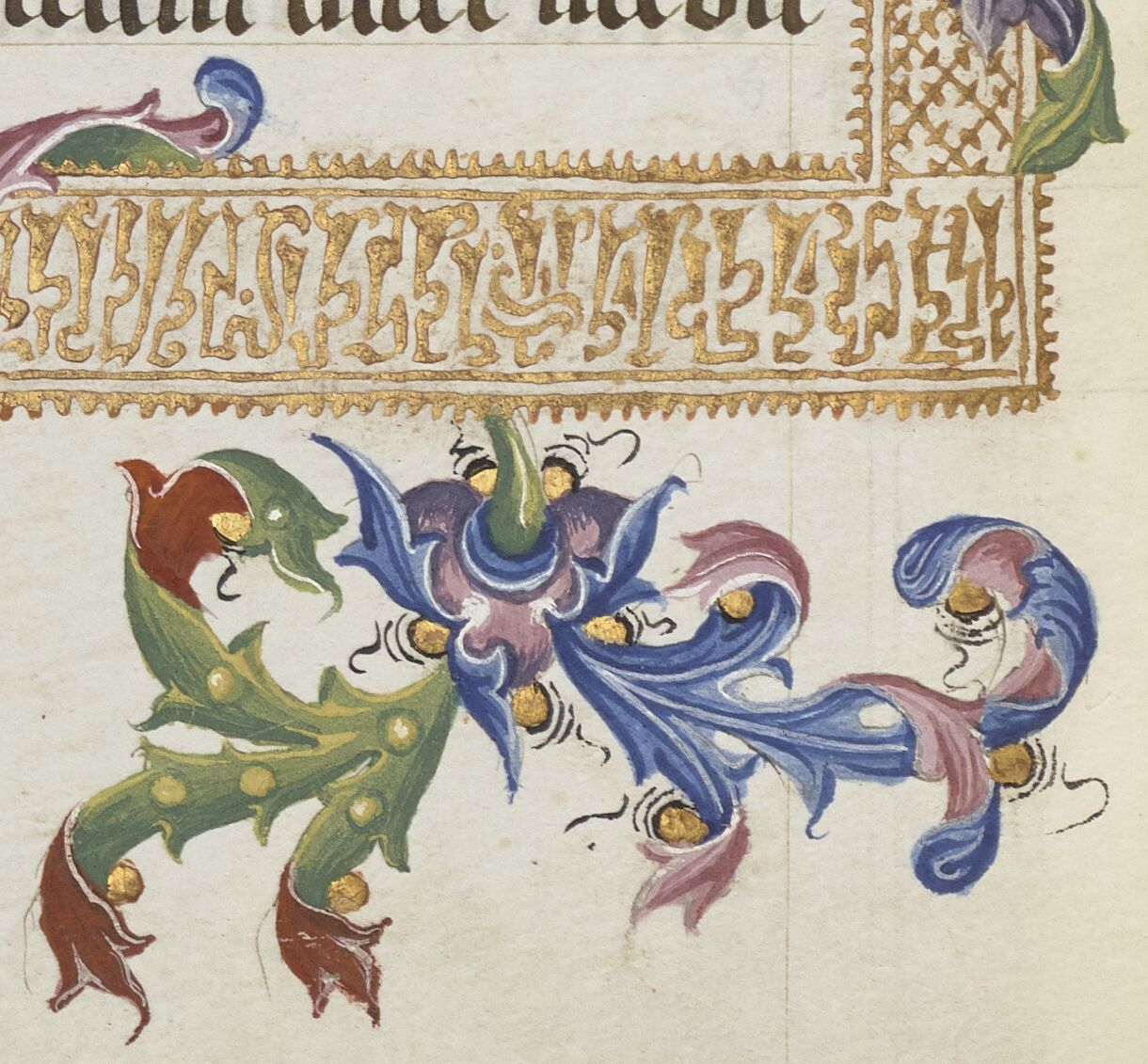This close-up photograph captures the intricate details of what seems to be a fragment of an ornate, illustrated manuscript or cloth tapestry. The central focus is a detailed and colorful, hand-drawn plant-like design. The plant features elongated, ribbon-like leaves in various shades of green, blue, and purple, accented with reds and yellows that resemble small bells. These swirling leaves, almost appearing to flutter, are beautifully detailed, creating a rich tapestry-like pattern.

Above this vibrant plant design, there is a meticulously laid out gold lace trim or border, featuring ornate rectangular and vertical gold elements that give a sense of elegance and symmetry. This gold pattern frames the plant design and adds a regal touch to the composition. The background, likely made of a hard material such as concrete or masonry, contrasts with the richness of the plant and gold designs.

The image conjures up a feeling of looking at the corner of an ancient, beautifully illuminated manuscript page, with elegant swirls, and gilt details that tell a story of artistry and craftsmanship from a bygone era. The finely detailed leaves and the ornate gold trimming hint at a blend of natural and artistic beauty, captured in this timeless close-up shot.